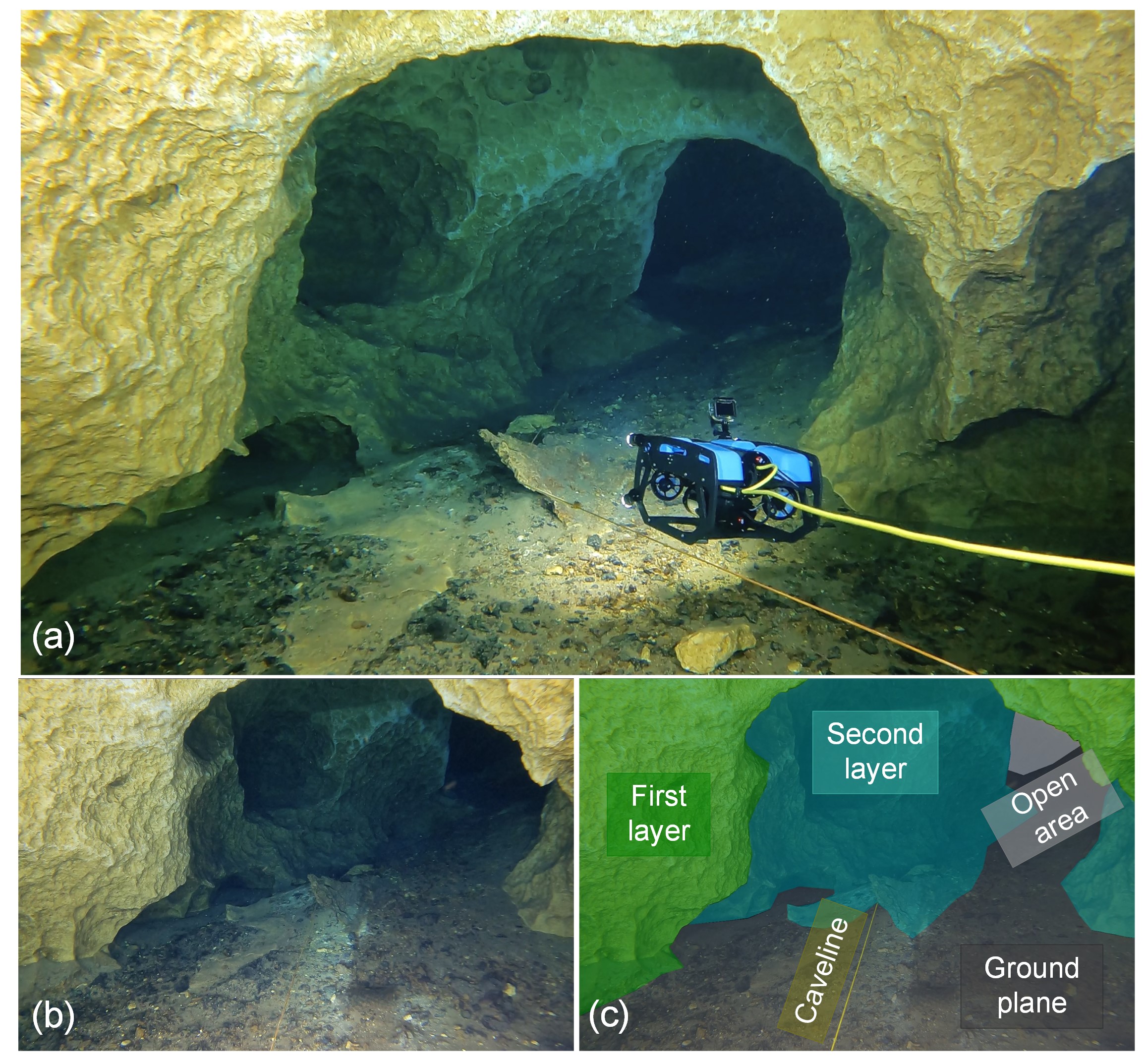The image is a square composite of three photographs, labeled A, B, and C, capturing different perspectives of an underwater cave. The largest photograph, occupying the top half of the composite (Box A), depicts a box-like blue underwater drone with a black frame and two large fans at its front and back, connected to a thick yellow wire. This drone, equipped with a small camera in a clear plastic case on top, is in the midst of being lowered into the shadowy, gray-green entrance of the underwater cave.

The bottom half of the composite displays two smaller photographs, divided equally. The bottom left photograph (Box B) shows the same cave entrance without the drone, emphasizing the shadowy, gray-green interior against the tan or gold exterior. The bottom right photograph (Box C) provides a labeled diagram of the cave interior, using various colors to denote specific features: layers, open areas, the ground plane, and the cave line. This labeling involves blue and green backgrounds, among other colors like pink, brown, and green, detailing the cave's stratigraphy and navigational elements. The overall composite offers a detailed exploration and analysis of the underwater cave, complete with visual aids and descriptive labels.